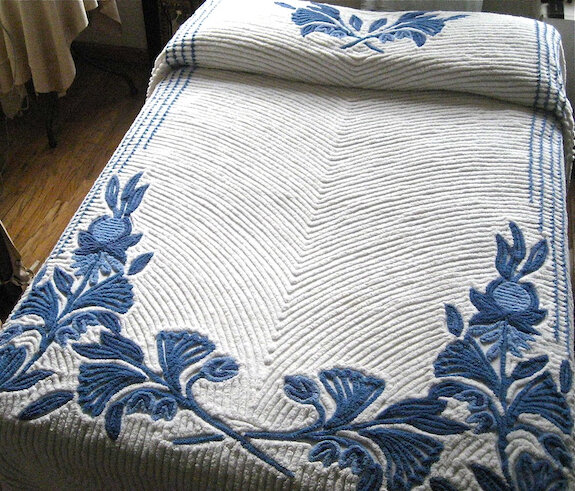This is a top-down view of a double-sized bed, impeccably made with a thick, heavily quilted white bedspread. The bedspread features intricate blue embroidery, with a crisscross pattern of large blue flowers and leaves at the foot and over the pillows at the head. The bedspread has distinct rows and lines, emphasizing its quilted texture. Flanking the sides of the bedspread are four embroidered blue lines. The bed is set upon a brown hardwood floor, adding warmth to the scene. In the background, off to the left, is an off-white curtain partially illuminated by soft, natural light filtering through a window just outside the frame. The overall composition captures the simple elegance and cozy ambiance of the bedroom.